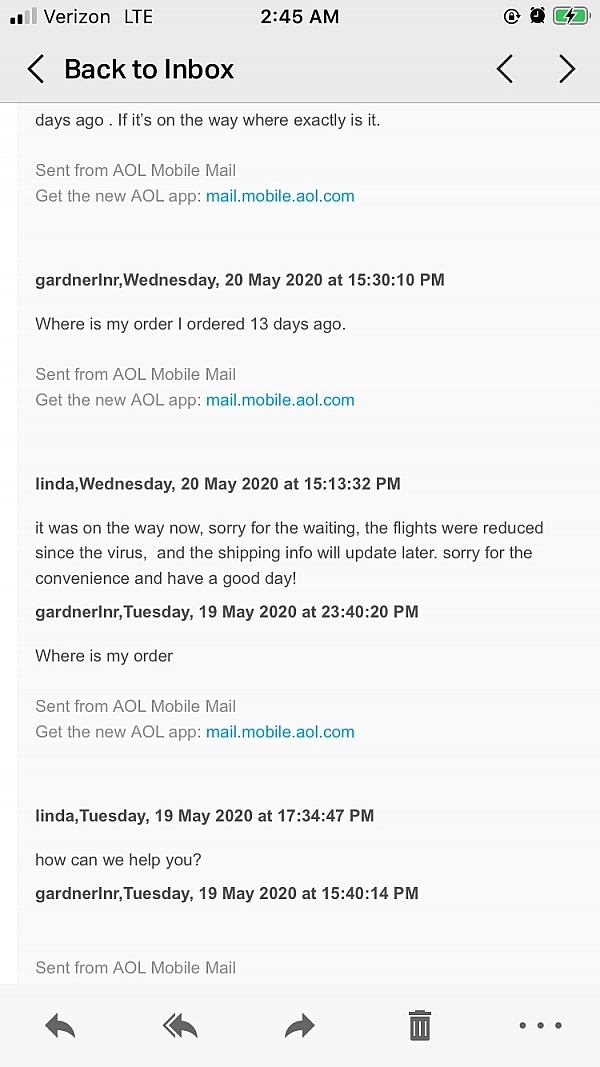The image features a rectangular, box-like shape filled with various pieces of detailed information. The content within the box includes an assortment of shapes and diverse lettering styles, forming different sentences. Scattered throughout the text are dates, numerical values, and times, providing specific details. At the bottom of this information box, there are several symbols, each indicating a unique function upon being clicked. Additionally, on the top right and bottom corners, there are distinct icons designed to offer users more options if needed.

The background of the image is predominantly gray, which contrasts sharply with the black letters, making the text easy to read. Interspersed throughout the information are blue hyperlinks, distinguishable by their color and their function of redirecting users to various other pages when clicked. Overall, the document exudes a highly informative aura, presenting a wealth of information in a clear and concise manner that is easy to digest.